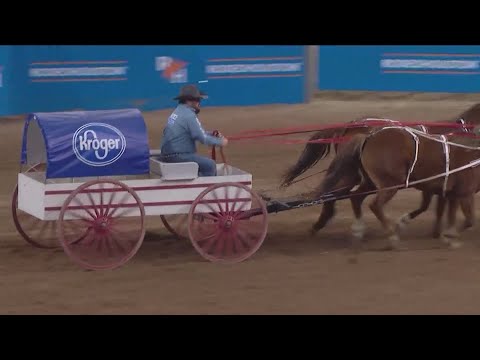The image captures a dynamic moment at a dirt-floor rodeo arena, framed by a cinematic-style black border on the top and bottom. A man, dressed in blue jeans and a gray shirt adorned with white lettering on the sleeves, is seated at the front of a simple, rectangular white wagon. The wagon has four red wheels, with the front pair being slightly smaller, and features a modest bench-like seat. The man holds red reins that control two dark brown horses. Behind him, a blue arched canopy displaying the white Kroger logo sits prominently on the wagon. The background is slightly blurred, showing banners with white and orange lettering and blue panel walls, suggestive of sponsorships and advertisements commonly found in a rodeo stadium.